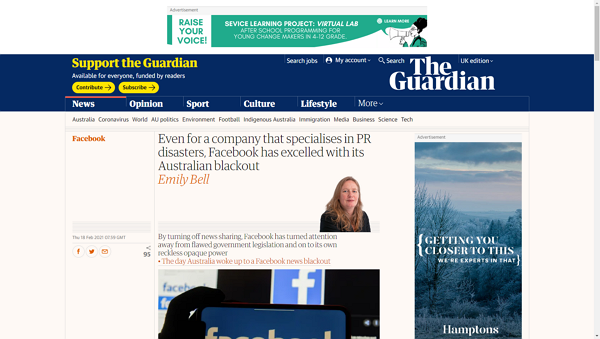The screen capture from The Guardian's website features an array of elements, starting with an overarching ad banner at the top. Set against a white background, the banner is predominantly green and showcases a cartoon illustration of a person with spiky black hair holding a speakerphone on the right side. The text on the left side reads "Raise Your Voice!" followed by "Service Learning Project Virtual Lab" in the center.

Below the advertisement is the website's own banner. In the top left corner, "Support The Guardian" is displayed in bold yellow font, accompanied by two clickable yellow buttons beneath it. In the top right corner is The Guardian's logo. Directly under the logo is a navigation bar with several menu tabs: "News" (selected), "Opinion," "Sport," "Culture," "Lifestyle," and "More" with a drop-down arrow.

The background color of the webpage is a subtle off-white. A vertical advertisement is positioned on the far right side of the page, featuring an image of a frost-covered forest. The text on the ad reads: "Getting You Closer to This. We're experts in that." and the brand name "Hamptons" is displayed at the bottom.

The main content of the webpage includes an article headline in bold black text: "Even for a company, the specialist in PR disasters, Facebook has excelled with its Australian blackout." This headline is attributed to Emily Bell.